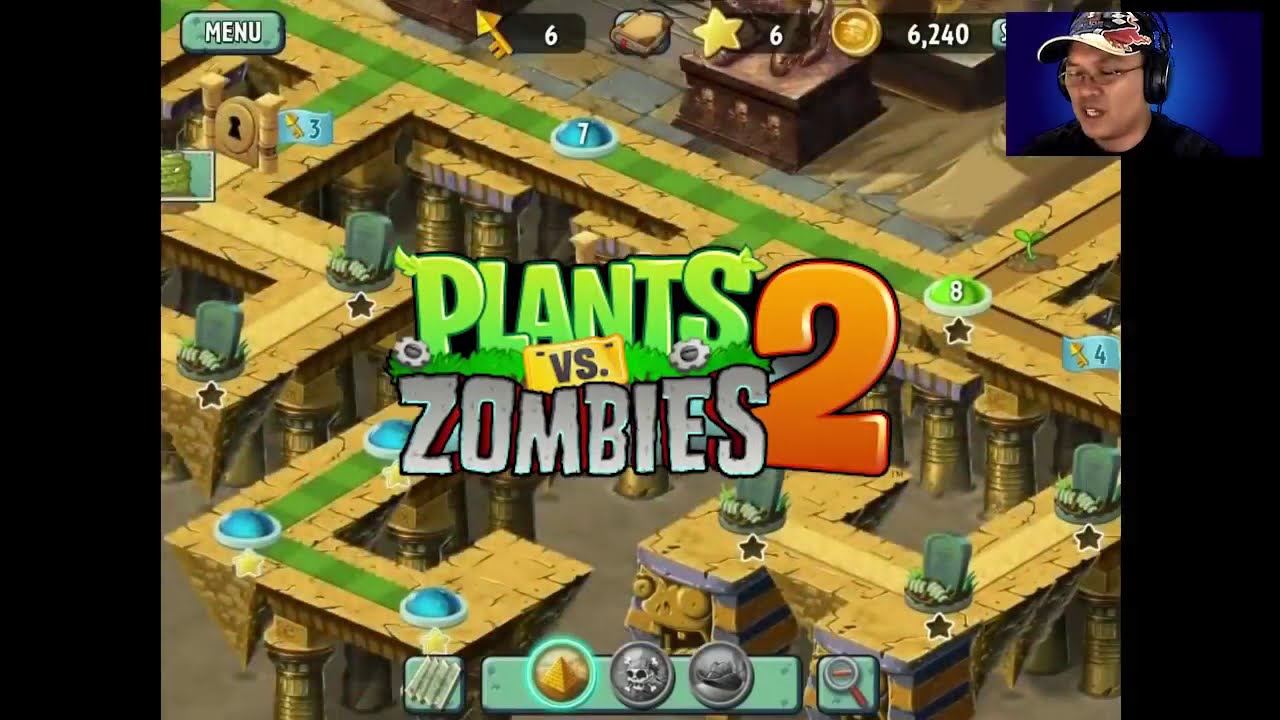The image depicts a screenshot from a streaming game channel, likely on YouTube, where a player is engaged in Plants vs. Zombies 2. The main portion of the screen features a desert-themed world select map with a series of pathways and nodes, resembling a maze. Some of these nodes are marked with gravestones. At the top left corner of the screen, the word "Menu" is prominently displayed. Accompanying this is an indicator displaying a pyramid icon with the number 6, a star icon also showing the number 6, and a money icon indicating a total of 6,240 coins. The bottom row features another menu with icons including a pyramid, crossbones, and a cowboy hat. In the top right corner, there is a webcam feed of the streamer, a white man around 30 years old, wearing a black t-shirt, a hat with a curved brim, over-the-ear black headphones, and glasses, set against a blue background, suggesting a Zoom window overlay. The map includes elements such as Egyptian-style carvings on stone pillars and partial views of statues in the cut-off section, enhancing the ancient, desert aesthetic.